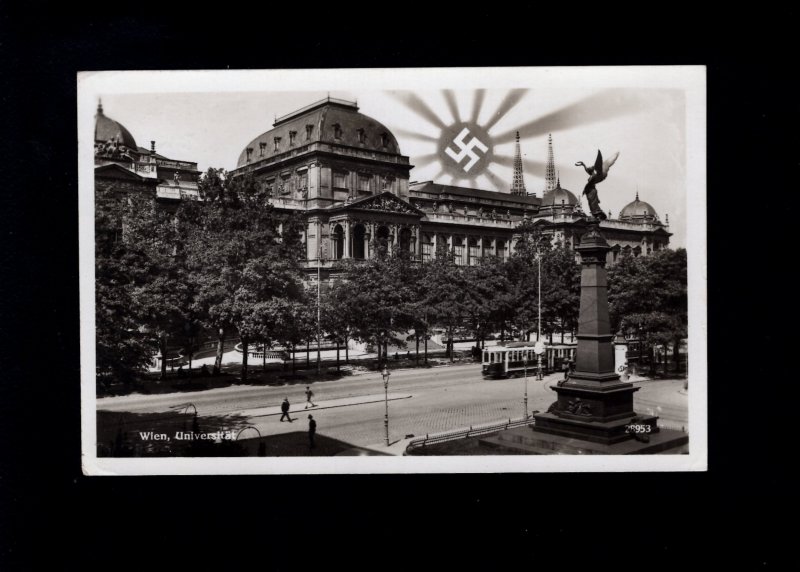This black-and-white photograph, tinged with a sepia tone, captures a chilling moment in history. Dominating the image is the stately presence of a large institutional building, likely a university, based on the small, white text found in the bottom left corner that reads "Wien University" (W-I-E-N-U-N-I-V-E-R-S-T). The setting is in Germany. The view is partially obscured by a line of trees, which stand between the building and a bustling street in the foreground. This street stretches diagonally from the bottom left to the right side of the photo and is dotted with pedestrians and a streetcar, emphasizing the everyday life of the period.

On the right side of the image, situated prominently in the foreground, stands a monument or obelisk topped with a statue that appears to have angelic wings. Above the university building, in the top right portion of the sky, a disturbing emblem demands attention: a dark, blurry circle resembling an inverted sun with dark rays extending outward and a white swastika, the notorious Nazi symbol, in its center. This ominous icon casts a dark shadow over the otherwise serene urban scene, marking the photo with a historical significance that's both haunting and poignant.